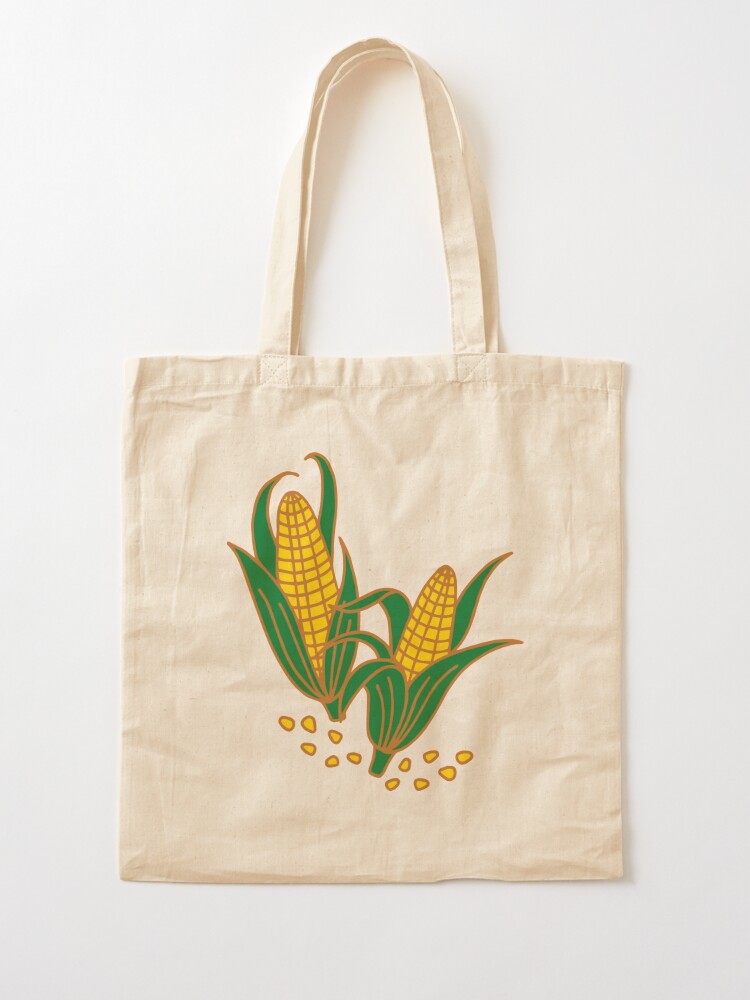This photograph features a reusable canvas shopping bag in a light taupe color, situated against a white background. The bag is characterized by its two long shoulder straps, sewn securely at the top on each side, facilitating easy carrying for shoppers. The lightweight, woven material of the bag appears very wrinkled, possibly indicating it is new or has been stored or shipped recently.

Adorning the front of the bag is a detailed, graphic illustration of two ears of corn, partially encased in their green husks with edges outlined in burnt orange. The left ear of corn has four leaves, while the right, slightly smaller ear has five leaves. Scattered in a path alongside the ears are twelve corn kernels, with six positioned symmetrically on each side. The bag, devoid of any text, enhances its simple yet elegant design, making it both functional and aesthetically pleasing for market errands. The bag's positioning in the image suggests it could be either hanging or lying on an unseen surface.